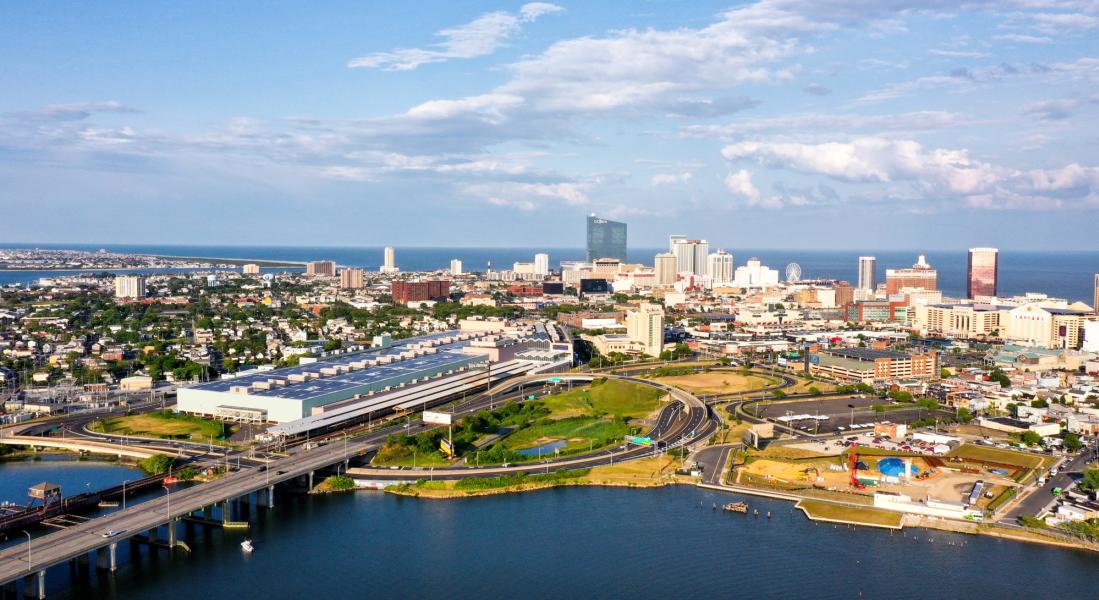This captivating image showcases an expansive cityscape from a high aerial vantage point, offering a panoramic view of the entire urban landscape. In the foreground, a glistening river flows through the city, highlighted by a prominent bridge on the lower left-hand side that connects different parts of the metropolis, hinting at robust infrastructure. The city itself is a blend of architectural styles, with towering high-rise buildings standing tall in the background, symbolizing commercial vigor, while the foreground is dominated by lower-rise, retro-style structures. The left side of the image is densely populated with both residential buildings and verdant patches, abundant with trees that add splashes of green. In the far background, the landscape extends into a vast body of water, suggesting the city might be situated on an island or a coastal region. The right side of the city appears more open and less densely constructed, offering a balance to the urban sprawl on the left. The entire scene is bathed in the warmth of a sunny day, with a clear, blue sky dotted with fluffy white clouds, creating an inviting and picturesque vista of this thriving, diverse metropolis.